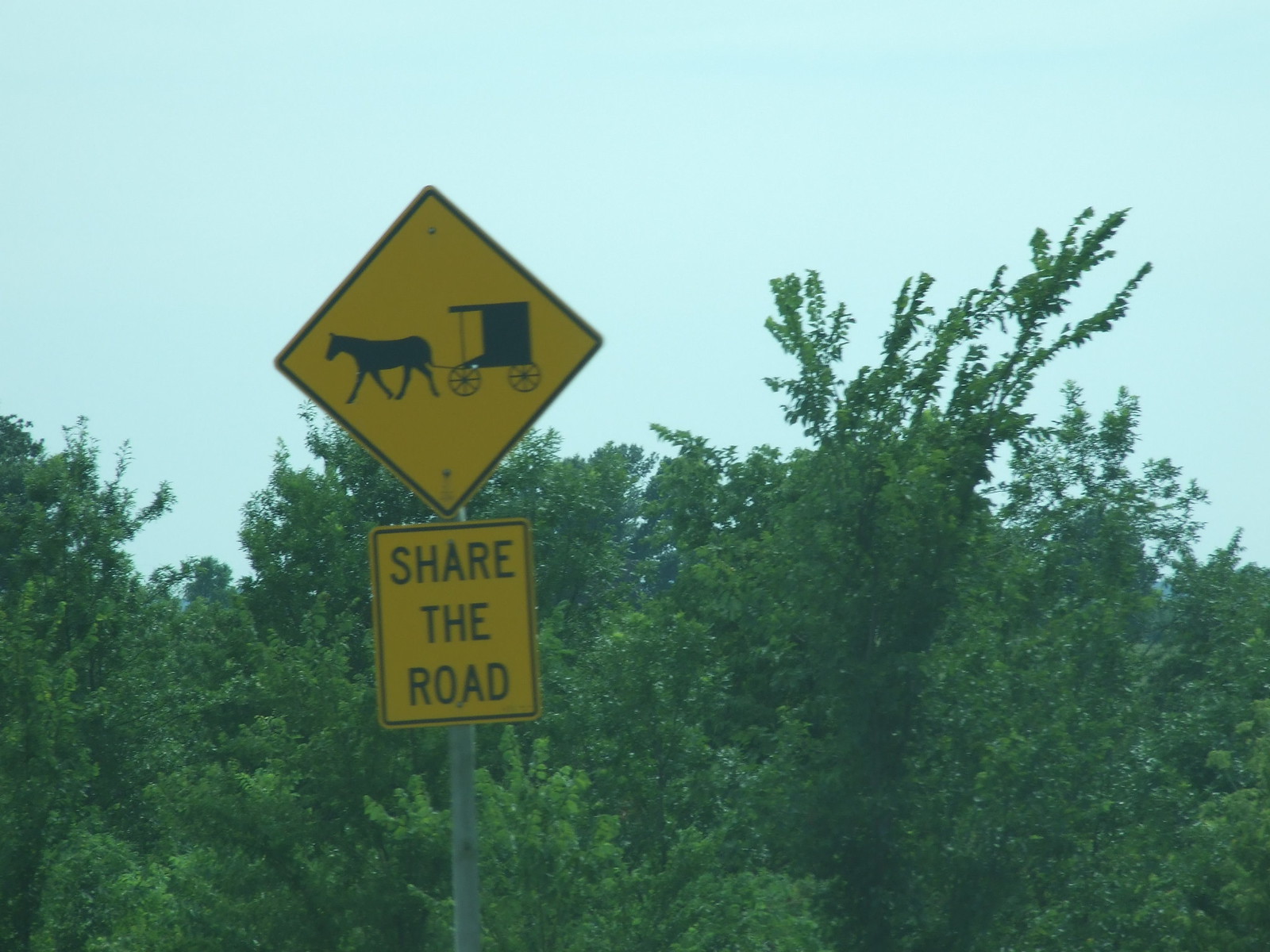This vibrant outdoor photograph captures a quintessential summer day where nature is thriving in full bloom. The lower half of the image is dominated by lush greenery; dense trees and thick shrubbery create a tapestry of vivid green hues that epitomize the essence of summertime. As your eyes ascend, the scene transitions into a serene sky painted in soft, light blue tones, providing a gentle contrast to the vibrant foliage below.

Positioned slightly to the left of center, a slender silver pole emerges from the bottom edge of the photograph, leading one's gaze upwards. Affixed to the pole is a bright yellow, square road sign that cautions with the message "Share the Road" inscribed in bold black letters. Just above this, another sign captures attention—a diamond-shaped warning sign depicting an Amish buggy drawn by a horse, also in black. The signs are slightly tilted, adding a touch of rustic charm to this peaceful rural landscape.